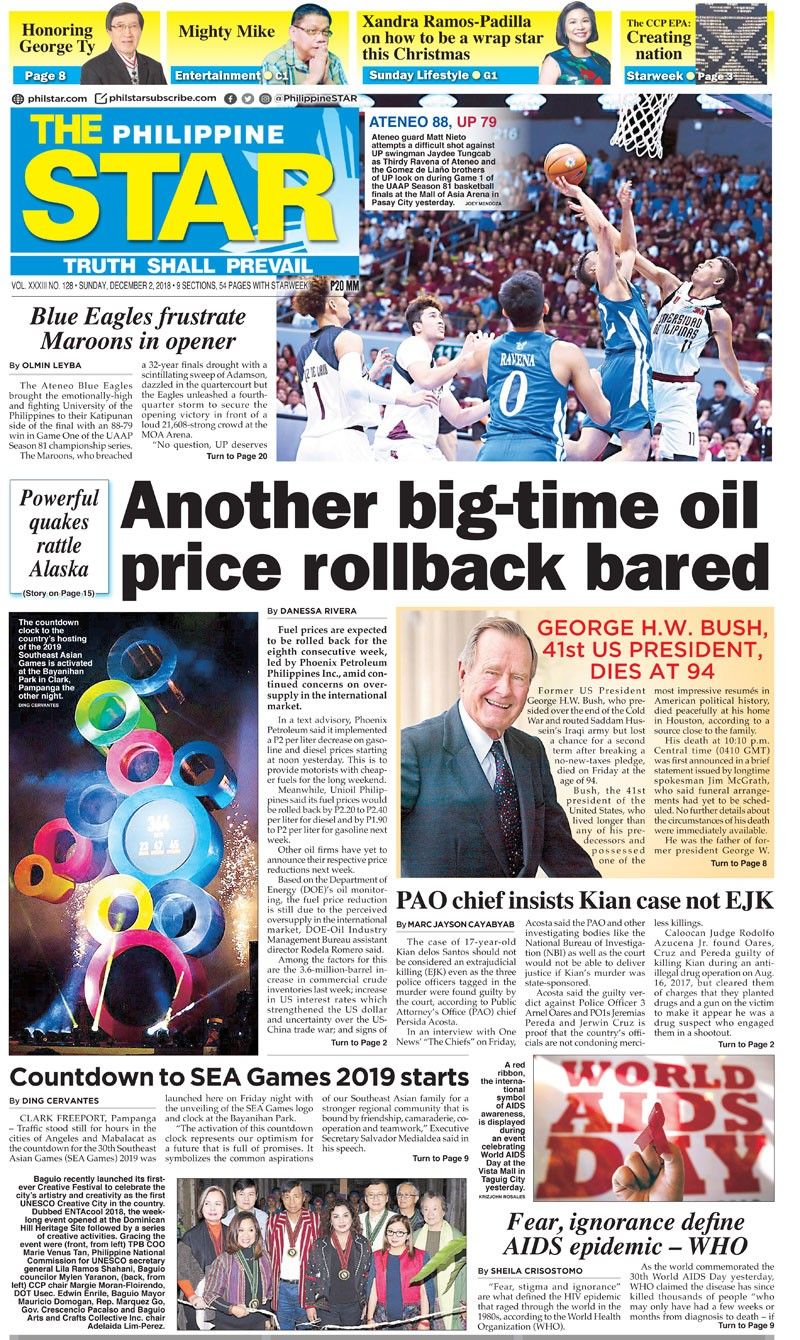**Front Page of the Philippine Newspaper - Detailed Descriptive Caption**

This image is a detailed screenshot of the front page of a prominent newspaper from the Philippines. The layout is vivid and information-rich, capturing various news highlights and special features.

At the top, we see several headlines against a distinctive yellow background. From left to right, the first headline reads "Honoring George Tai," accompanied by an image of a gentleman with black hair and glasses dressed in a black suit. This content is found on page 8. Next to it is the headline "Mighty Mike," featuring an older gentleman with glasses wearing a blue and white striped shirt.

The entertainment section highlights "Sandra Ramos Padilla on How to Be a Rap Star This Christmas" with her stylish image. Sandra is a fashionable woman dressed in a blue dress with a floral pattern, and she has short black hair. This feature is located in the Sunday Lifestyle section, page G1.

Following that is another headline about "The CCP EPA Creating Nation Star Week," illustrated by a striking black image adorned with geometric designs.

Dominating part of the page is the prominent logo of the newspaper, "Philippine Star," placed on a blue background. The words "Philippines" are bold in white text below it, suggesting the newspaper's broad focus.

Beneath these sections is a dynamic image of a basketball game, showcasing players in white and blue uniforms. One of the players is captured in action, attempting a dunk. The scoreboard shows Ateneo leading with 88 points against UP’s 79.

Below the sports section is a major headline in bold black text, declaring "Another Big Time Oil Price Rollback Bared," signaling significant economic news.

An adjacent smaller box with red text on an orange background announces the death of George H.W. Bush, the 41st U.S. President, who passed away at the age of 94. This is paired with a respectful image of George H.W. Bush.

This front page intricately weaves together stories of celebration, lifestyle, sports, and significant global news, providing readers with a comprehensive and engaging view of current events.